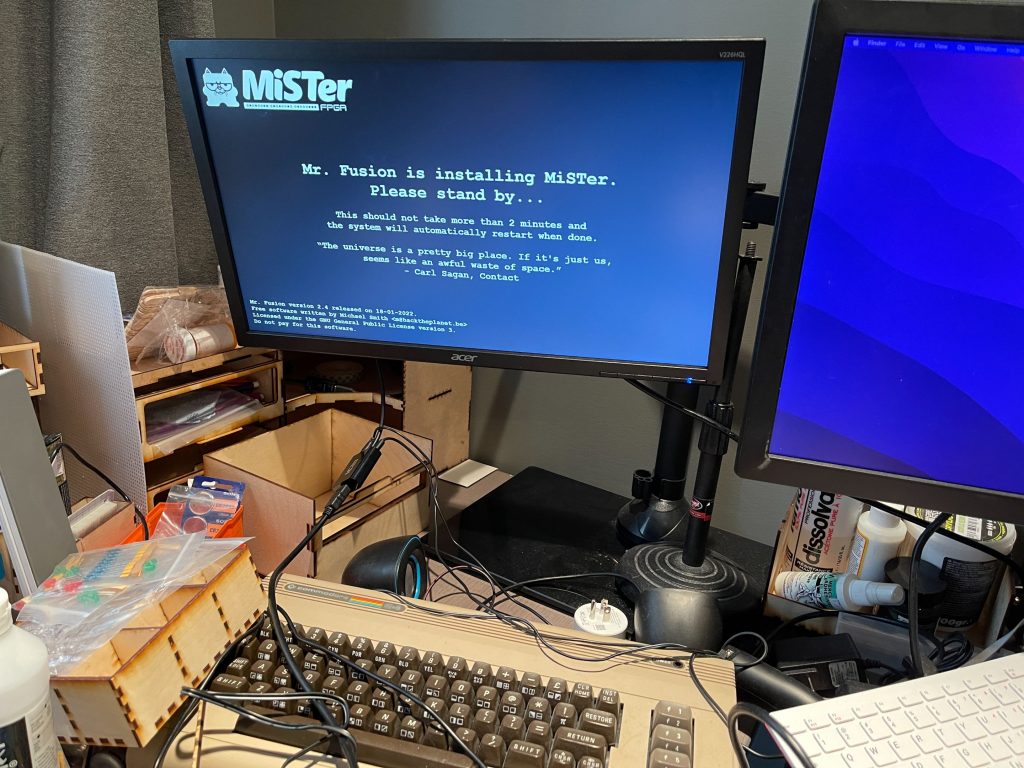This photograph depicts a cluttered office area with a desk featuring two computer monitors and two keyboards. The larger monitor on the right displays a plain blue background, while the smaller monitor on the left shows the phrase "Mr. Fusion is installing Mr. Please stand by. This should not take more than two minutes. The system will automatically restart when done." Additionally, it includes a message from Carl Sagan’s Contact: "The universe is a pretty big place. If it's just us, it seems like an awful waste of space." There is also a small cartoon animal symbol to the left of the word "Mr." The desk is strewn with various office supplies, including bottles and wires. The modern white keyboard is positioned below the larger screen on the right, and a much older keyboard with a yellowish tint and outdated keys sits in the middle-left of the desk. Numerous black wires and plugs run across the area, further contributing to the messy appearance.